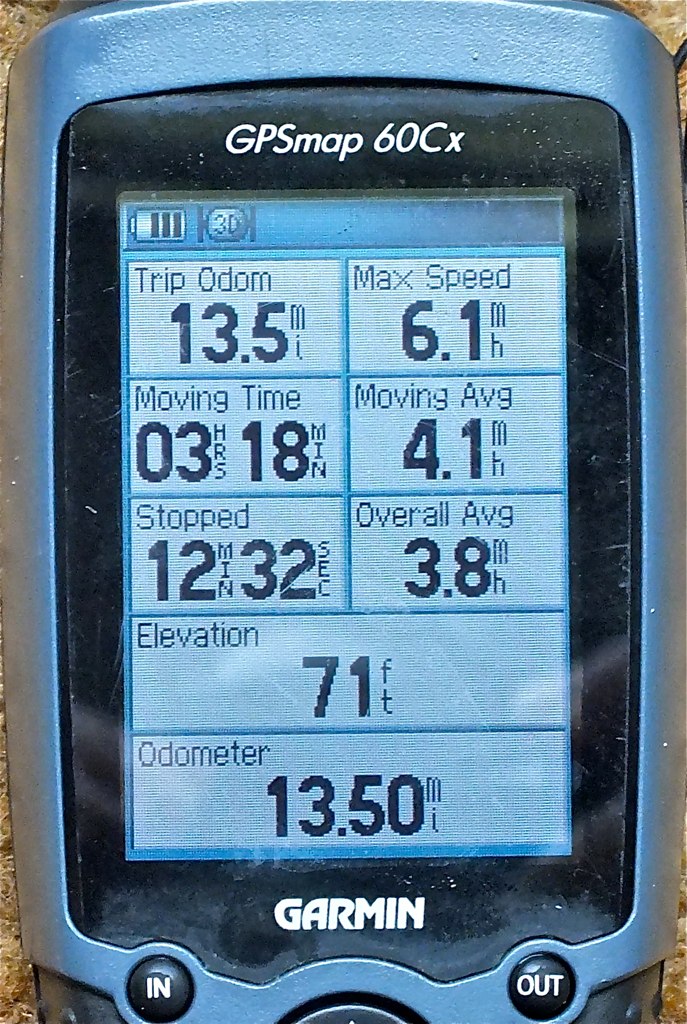This close-up image showcases a Garmin GPS device, specifically the GPS Map 60CX model, used to track various travel statistics, potentially for a business monitoring driver routes and performance. The outer rim of the device is silvery blue, framing a black square that prominently displays the brand name "Garmin" in white print. Just below the Garmin label, and flanking it to the left and right, are the words "In" and "Out." The digital display at the center presents a wealth of detailed information:

- **Battery Status**: 75% charged, indicated by three out of four bars.
- **GPS Mode**: Displaying a "3D" signal status.
- **Trip Odometer**: 13.5 miles traveled.
- **Maximum Speed**: 6.1 mph.
- **Moving Time**: 3 hours and 18 minutes.
- **Moving Average Speed**: 4.1 mph.
- **Stopped Time**: 12 minutes and 32 seconds.
- **Overall Average Speed**: 3.8 mph.
- **Elevation**: 71 feet above sea level.
- **Total Odometer**: Consistent with the trip odometer at 13.50 miles.

The device's display succinctly encapsulates critical travel data such as distance traveled, time spent moving, and stationary periods, offering comprehensive insights for managing and monitoring driving activities.